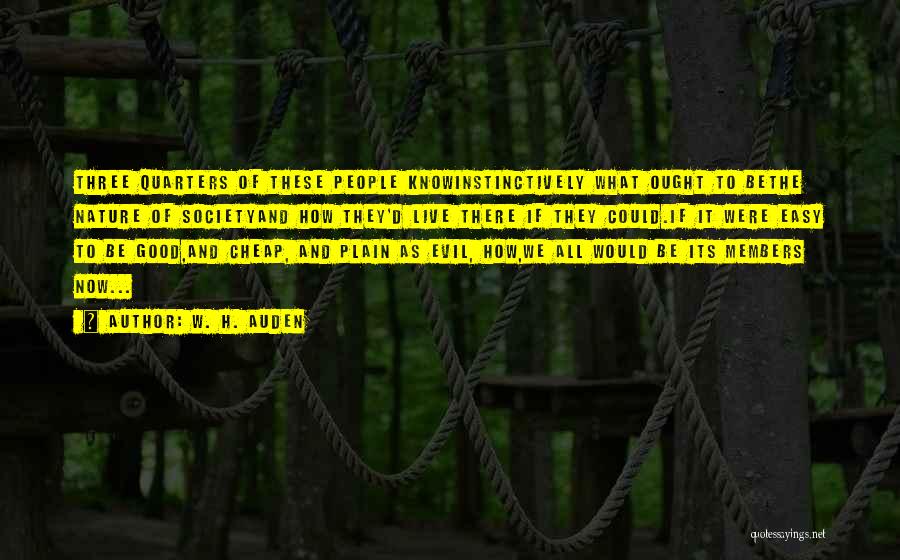The image depicts a high adventure ropes course set in a dense forest, characterized by a dark filter. The structure features a lattice framework with wooden poles and hamstrings intertwined, creating platforms and hanging ropes for climbing and ziplining activities. Superimposed on this background is a piece of text presented in black on yellow lines. The text reads: "Three-quarters of these people know instinctively what ought to be the nature of society and how they'd live there if they could. If it were easy to be good and cheap and plain as evil, how we all would be its members now...?" This quote, authored by W.H. Auden, is framed by yellow banners, making it stand out against the forest setting.